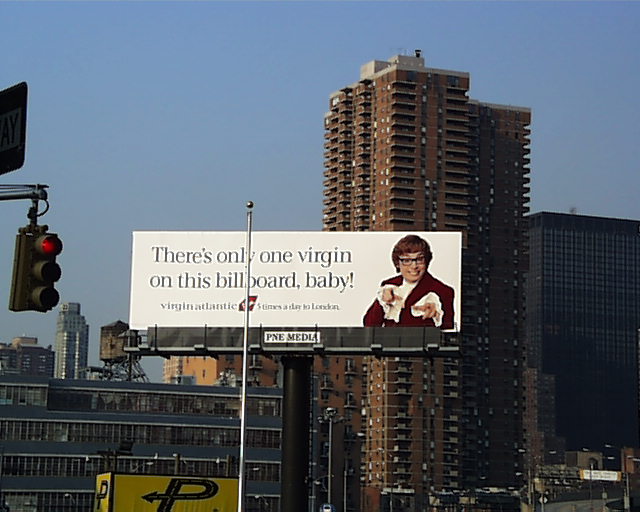In the heart of a bustling cityscape under a clear blue sky, a prominent billboard advertising Virgin Atlantic Airlines captures attention. The billboard, featuring the iconic Austin Powers character, played by Mike Myers, proudly displays the cheeky tagline, "There's only one Virgin on this billboard, baby! Virgin Atlantic. Five times a day to London." Austin Powers, seen with his recognizable glasses, short dark hair with bangs, and a smile, stands out against a vivid background. Below the tagline, the name "PNE Media" is noted. Encircling the billboard is an urban panorama with multiple high-rise buildings, including one that appears to be an apartment or condo, showcasing numerous glass windows. A stoplight, turned red, hangs over the frame from the left, hovering above a one-way sign that's partially out of view. Dominating the lower left side is what seems to be a truck or parking garage with a distinct black "P" on a yellow background. Additionally, a tall flagpole stands sentinel in front of the billboard, devoid of any flag. Streetlights dot the scene, completing the quintessential city view.